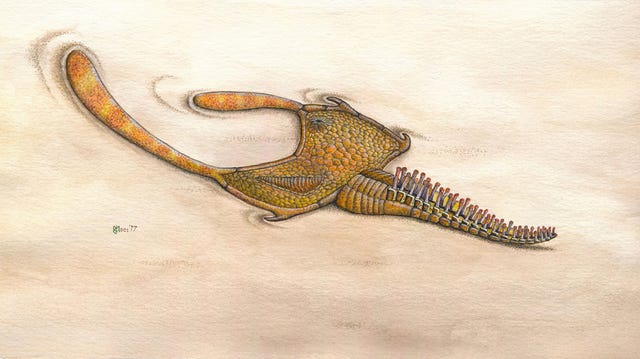The image is a painting depicting an abstract life form lying in the sand. The creature has a prominent spine on its back, resembling a tail, and a flat, heart-shaped front. It's primarily green, with a texture akin to snakeskin, and features semi-striped ear-like protrusions. The life form appears dried out and possibly dead, hinted by its brownish tones and the way it's positioned, suggesting an upside-down state. Its surroundings show signs of movement, indicating some form of recent locomotion that disturbed the sand. The painting's background is a soft, neutral eggshell color, adding to the textured and slightly eerie feel of the artwork. The artist's signature can be seen toward the bottom left of the image.